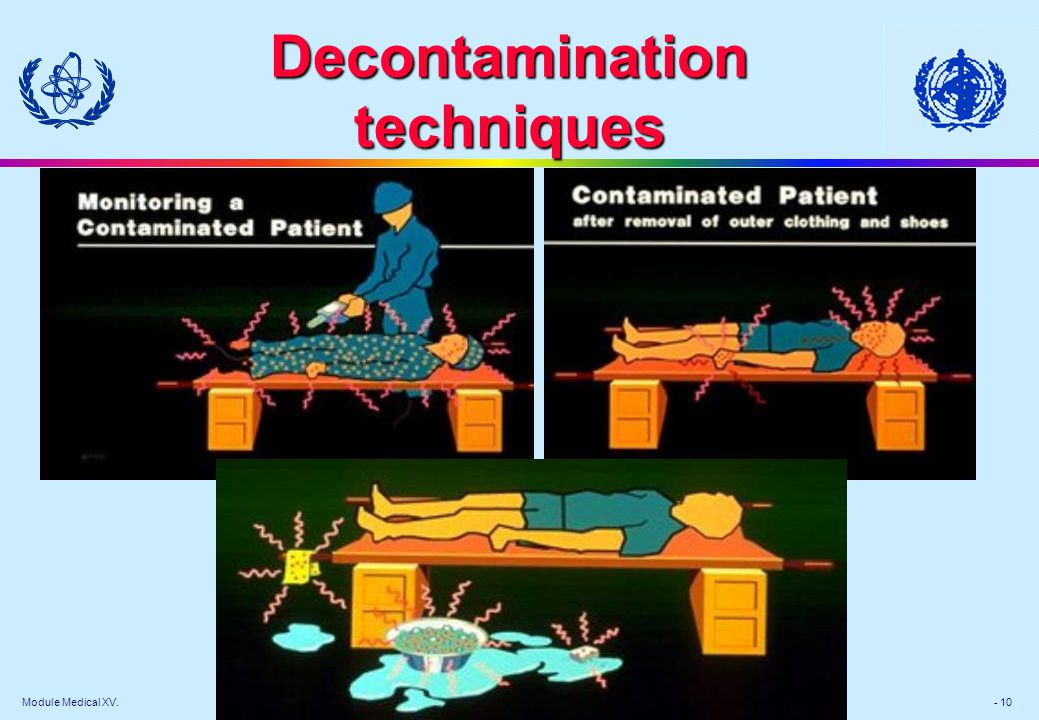The light blue poster titled "Decontamination Techniques" in bold red lettering is centered at the top, flanked by two blue logos on either side. Each logo features a string of leaves, resembling a wreath, and unique symbols: an orb-like figure and a globe intertwined with wheat stalks. Below the title, there are three clipart-style images set against a green background, depicting the decontamination process in steps.

The first image, labeled "Monitoring a Contaminated Patient," shows a person lying on a makeshift cot, in a blue nightgown with polka dots and small red curly cues indicating contamination. A technician in a blue suit and hard hat is scanning the person with a device.

The second image, titled "Contaminated Patient After Removal of Outer Clothing and Shoes," depicts the same person now wearing only boxer shorts and a t-shirt, showing fewer red curly cues.

The third image, which has no wording, illustrates the final step. The person is no longer visible, but there is a blue and white bowl and a puddle of water on the floor, signifying that the contamination has been fully removed and contained.